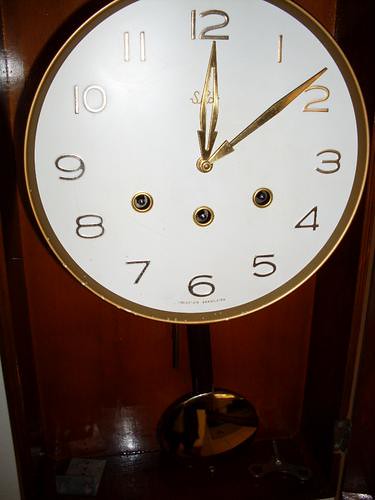This close-up photograph captures the intricate details of the interior front panel of a majestic grandfather clock. The casing is crafted from richly polished mahogany, its deep, dark hues exuding a blend of brown, reddish, and subtle purple tones. Dominating the upper portion of the frame is the large, round clock face, encased in a refined gold frame. The clock face, free of lines or markers, is adorned with elegantly styled gold numerals. The time displayed is approximately 12:08, with the slender, pointed clock hands also rendered in gold. Below this commanding clock face, a gracefully suspended pendulum glints with a matching golden finish, further validating the timepiece as an iconic grandfather clock. The photograph not only showcases the aesthetic allure but also hints at the precision craftsmanship involved in its making.